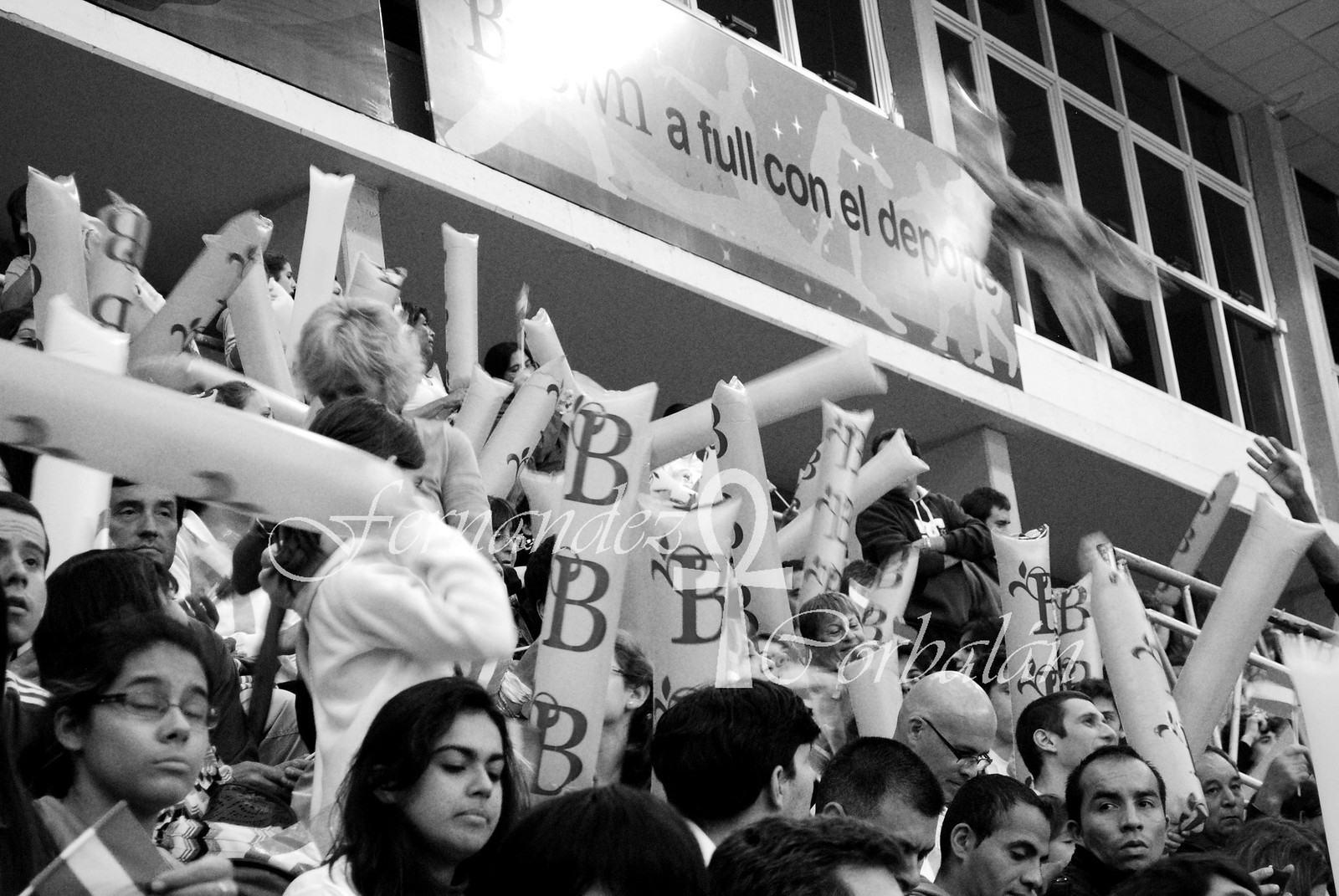This black-and-white photo captures an indoor setting with a tiled ceiling above and rectangular windows in the background. The image shows a diverse group of men and women seated on bleacher-style seating, with metal railings along the sides. The attendees are holding light gray, inflated tubes, many of which have the capital letter "B" repeatedly printed on them. Above the crowd is a poster with black writing in what appears to be Spanish or Portuguese, and cursive white text that looks like a name, possibly "Fernandez" followed by "por balan." There is also a flag being held up by one of the people. The scene seems to be at a lively event, likely involving students, who are looking in various directions, adding to the dynamic feel of the moment captured.